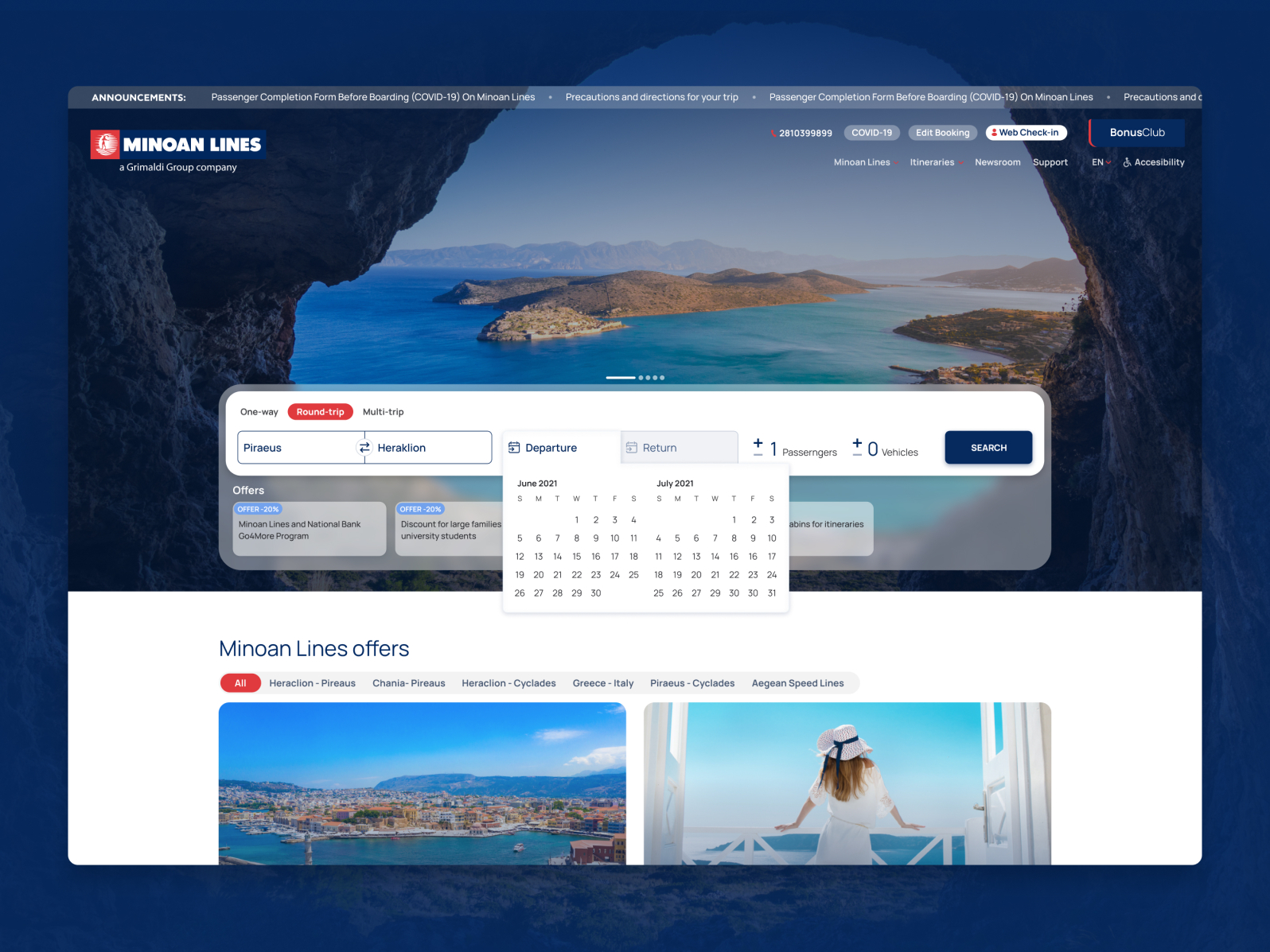A detailed caption for the image could be:

"The image appears to be a screenshot of a travel company's website specializing in vacations to an island nation. The background is a picturesque photograph taken from within a cave, offering a stunning view of a set of lush islands surrounded by a brilliant blue ocean. At the top of the website, an announcement bar displays several options such as 'COVID-19,' 'Web Check-in,' 'Bonus Hub,' accompanied by a calendar for selecting departure and return dates, suggesting features for ease of booking. Below this, there is a navigation section that includes options like 'Round Trip' and other promotional offers. 

Central to the image is a cityscape of an idyllic island city, juxtaposed on the right side by a serene photograph of a woman in a sundress and white hat with a blue ribbon, leisurely looking out at the ocean from a balcony. Behind her stand two open white French doors, adding to the vacation appeal. The overarching cave photograph in the background has been artistically zoomed and darkened with a blue overlay to complement the website's inner images, ensuring a coherent visual theme that enhances the travel website's allure."